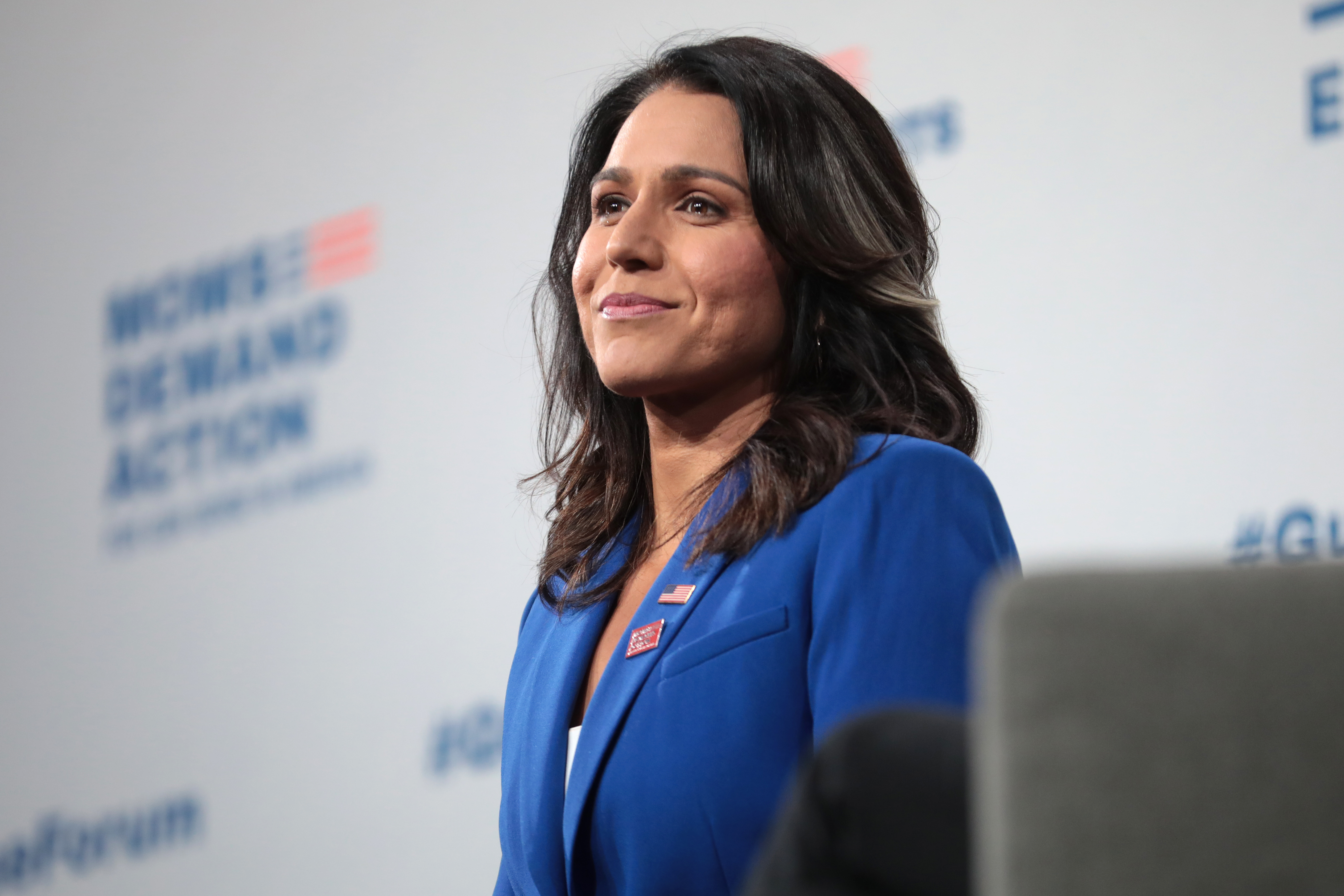In the photograph, a confident woman who appears to be in her 40s is seen from the chest up, angled slightly to the left. She has shoulder-length dark hair, almost black, and she is wearing a blue business casual jacket with a pocket on her chest. On the left lapel, there are two pins: a small American flag pin on top and a red resin pin with unreadable writing beneath it. Underneath the jacket, she sports a white top. The woman, with a smile on her face and slightly tanned skin, exudes a political aura. In the blurred background, there's a press banner that is predominantly white with blue text, featuring the phrase "Women Demand Action" and some red stripes as part of the logo. In the bottom right corner, a gray square object with black elements peeks into the frame, adding depth to the scene. The backdrop and her poised expression suggest she may have just delivered a speech at a political rally.